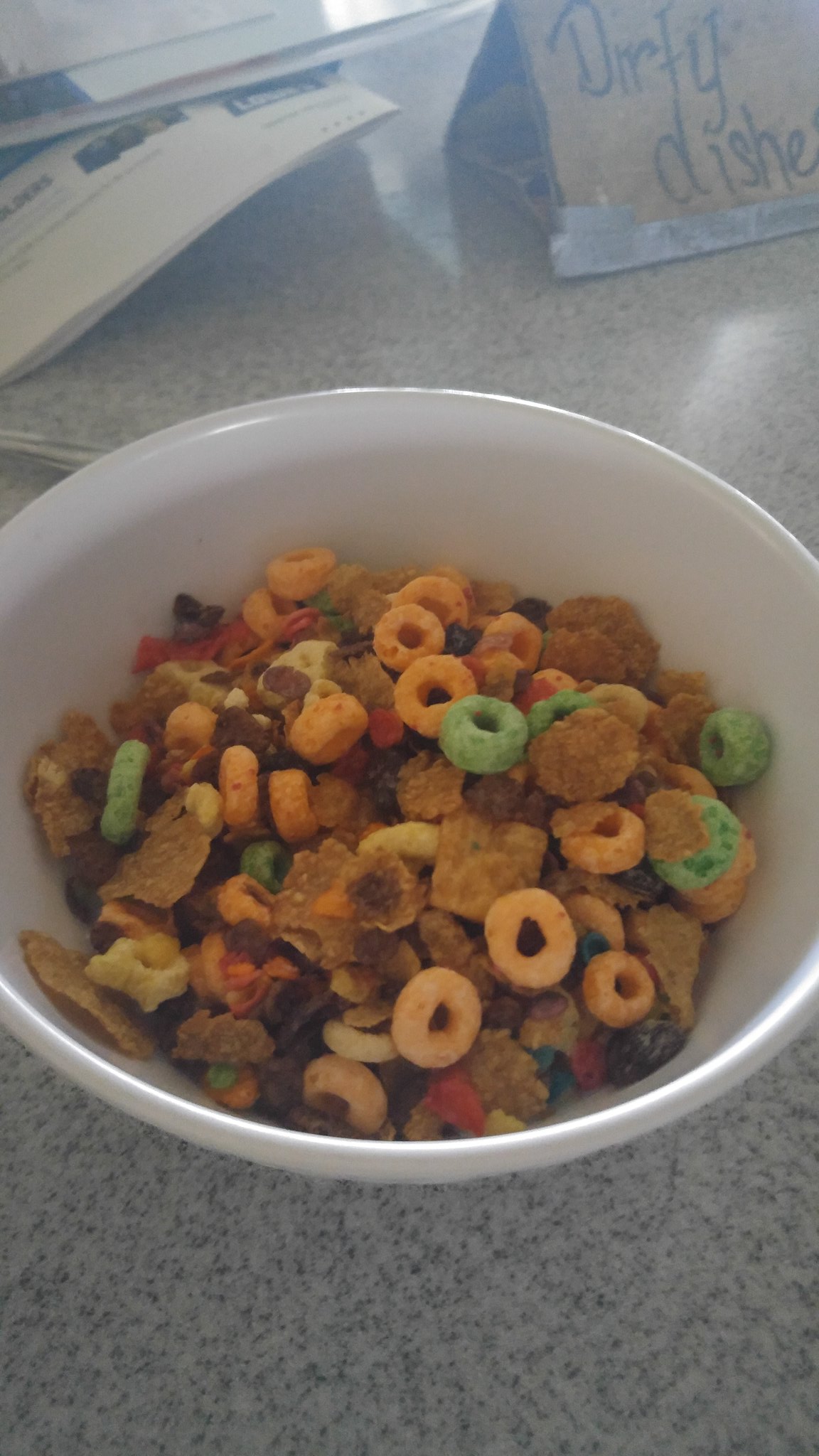The image features a white bowl filled with a mixture of various cereals, sitting on a white and black speckled or marble-like kitchen countertop. The bowl contains several types of cereal including colorful loops resembling Froot Loops or Apple Jacks, flat flakes that could be Corn Flakes or Wheaties, square pieces that might be Chex, and irregularly shaped honeycomb-like cereal bits. There is also a mention of raisins being present. No milk is in the bowl, making it dry cereal. In the background, there is a triangular, handwritten sign made from cardboard that says "Dirty Dishes" in black marker. To the left of the sign, a stack of mail, newspapers, catalogs, or possibly a cookbook can be seen. The image is rectangular and has a vertical orientation. The countertop is predominantly gray and white, and there is no spoon in the bowl.